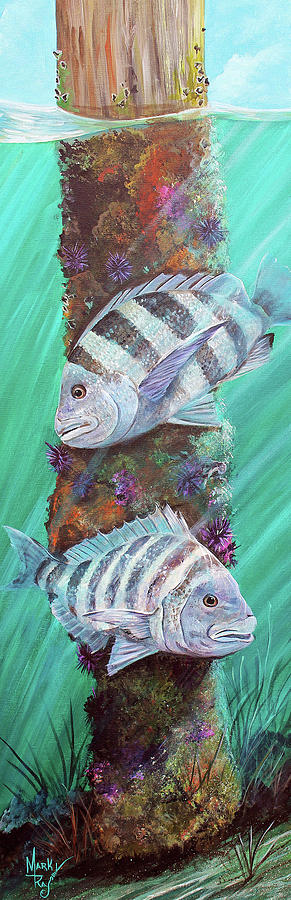An illustration-style image depicting an underwater scene is signed in teal by the artist in the lower corner. The ocean floor is covered with grainy, gray sand and sparsely dotted with bits of plant life. Two large fish, adorned with black stripes and shaded in hues of light blue, navy, and white, swim gracefully in front of a pole extending through the center of the water. This pole is encrusted with various forms of vibrant marine flora, including purple, blue, and green vegetation, and features a striking, spiky purple flower. Near the top of the pole, pink plant life can be spotted alongside patches of brown and green algae. The water around them is a clear turquoise, and peeking through the surface, a glimpse of blue sky peppered with fluffy white clouds adds a serene backdrop to this underwater tableau.